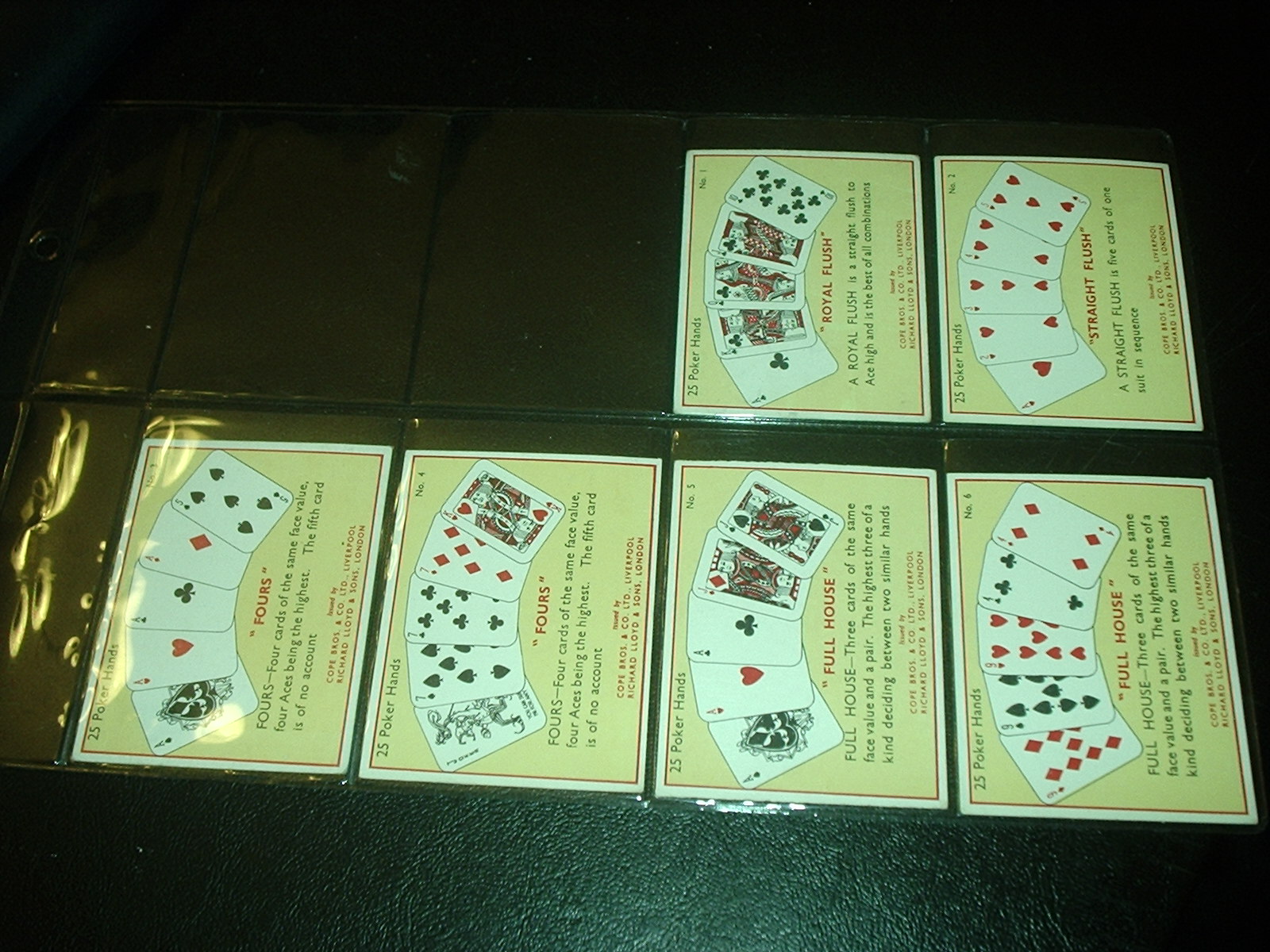The image captures a collection of various poker hand advertisements, neatly displayed on small signs or placards, each illustrating a different poker hand. The signs are slightly tilted to the side, making them somewhat challenging to read. 

In the bottom row, there are four placards:
1. The first placard demonstrates the poker hand known as "Fours," showcasing a set of four cards.
2. The second placard also displays the "Fours" hand, identical to the first.
3. The third placard illustrates a "Full House" poker hand.
4. The fourth placard again demonstrates a "Full House" hand.

Above this row, two more placards are placed:
1. One sign features the highest-ranking hand, a "Royal Flush," with the corresponding cards displayed.
2. The other placard shows a "Straight Flush," accompanied by the set of cards that form this hand.

Each placard is set against a creamy white backdrop with a spread of playing cards displayed prominently. Below each spread, there is a black font description detailing the specific cards that make up the hand, providing a clear and informative guide to identifying these common poker hands.